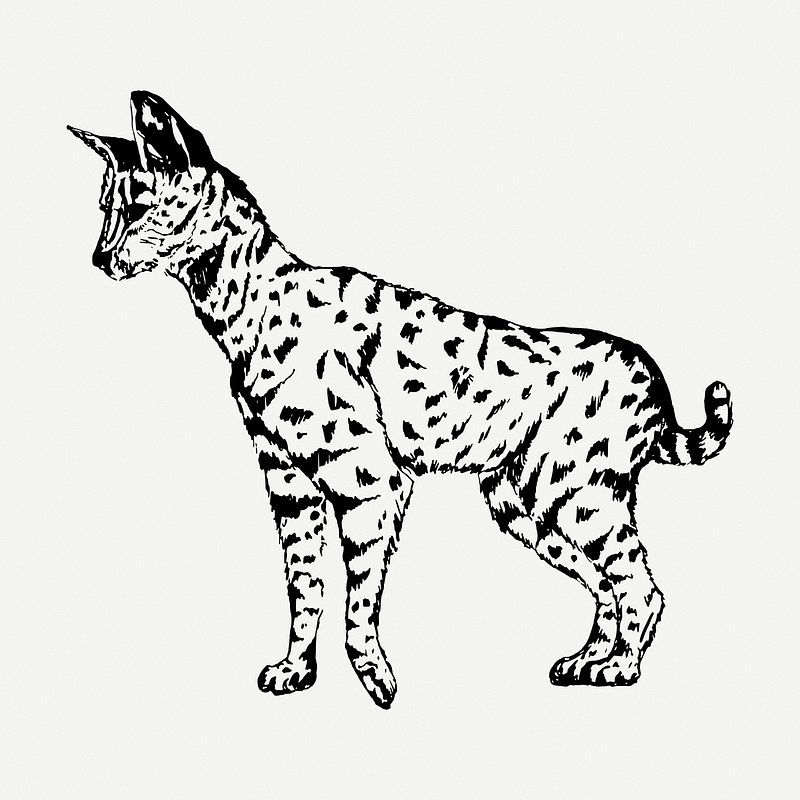This black-and-white woodcut-style illustration features a small wildcat set against a contrasting white background. The cat’s body is decorated with black patterns that resemble a mix between stripes and small rectangular markings. It stands with its back hind legs close together while its front left paw is slightly raised, suggesting a paused motion, and its right paw remains grounded. The cat is facing left, appearing to have its attention captured by something off to the side. The short, stumpy tail is patterned with alternating black and white stripes, and its ears are large, conical, and perked up, adding to its alert demeanor. The head is proportionately small with a pointed nose, and thick neck, with black stripes running from the forehead down towards the nose. The overall stance and forward-pointed nose emphasize its focused and attentive nature.